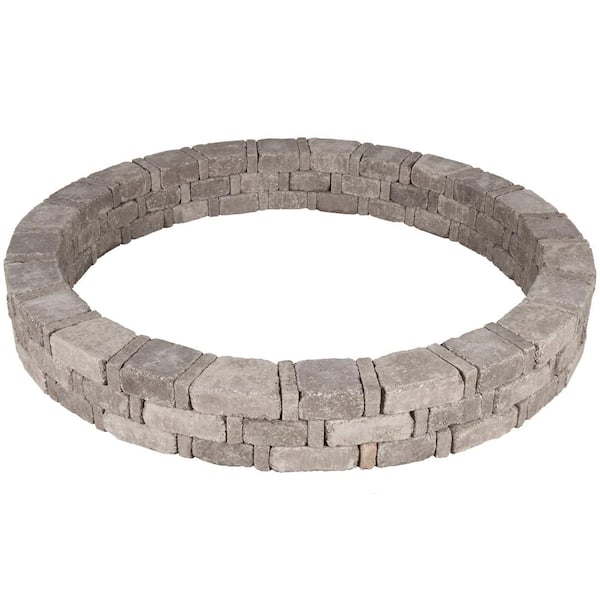The image features a large circular stone ring set against a very plain white background. The ring, which appears to be about 50 feet in diameter, is constructed from interlocking gray stone blocks arranged in a meticulous pattern. The structure consists of three levels or layers of stone blocks. Each level alternates between square blocks and longer rectangular blocks, creating a visually striking interlocking design. The blocks on each subsequent layer overlap with the ones below, forming a cohesive and sturdy pattern throughout the entire structure. The center of the circular ring is empty, devoid of any additional elements or text. Overall, it showcases a sophisticated and uniform brickish gray stone design.